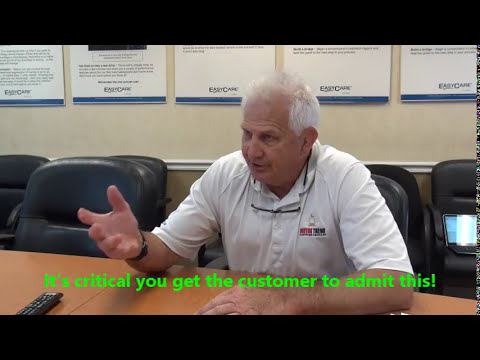The image depicts an older, balding white man with thinning white hair, seated at a large brown wooden conference table in a business conference room. He is wearing a white collared polo shirt adorned with red and black text and possibly a bird logo on the left breast. The man has glasses strung around his neck and is in the midst of speaking, his right hand raised while his left forearm rests on the table. His posture and expression suggest he is conveying an important message. Surrounding him are several black leather office chairs and visible on the table is a black remote control. Behind him, on a beige wall, are several white and blue posters and on the chair to the far right, an open laptop is visible. The scene is framed horizontally with black bars at the top and bottom. In neon green text across the image, it reads: "It’s critical you get the customer to admit this!"